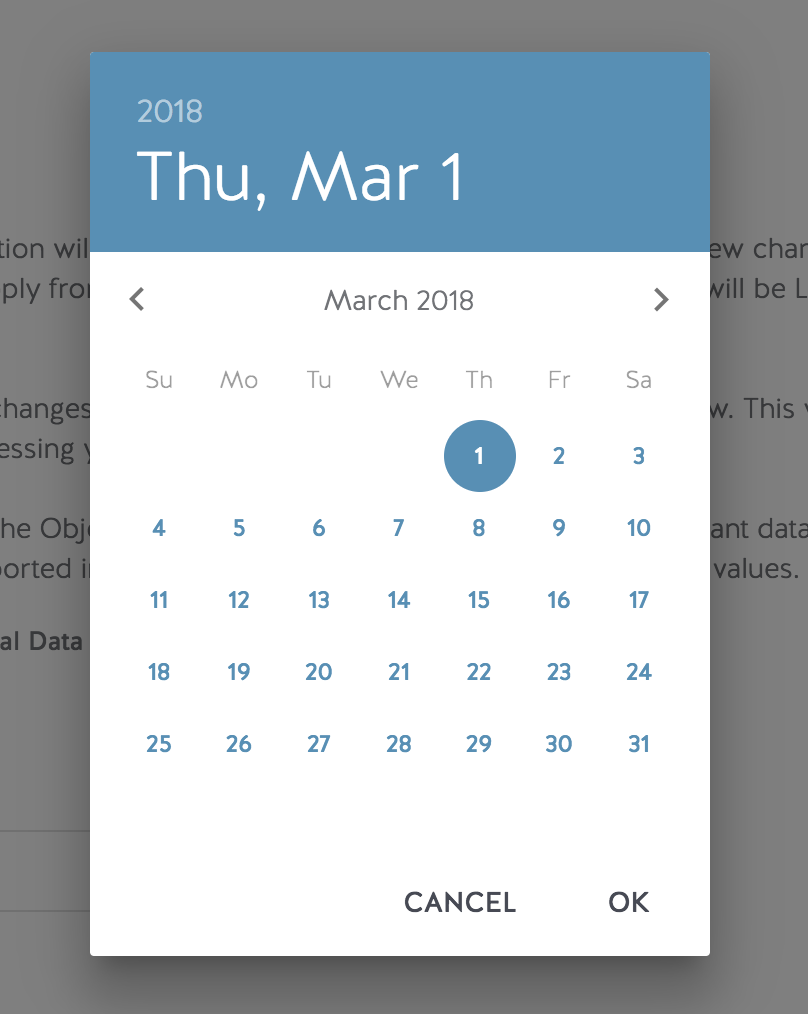In the background of the image, there is a page filled with text, displaying words like "new," "change," "changes," and "data values," although the text is not entirely legible. The foreground prominently features a pop-up calendar from the year 2018. The calendar is open to Thursday, March 1st. Navigation arrows are present: a left arrow to revert to January and a right arrow to advance to December. The current month, March 2018, is centered at the top of the calendar. Below, the days of the week are abbreviated (S-U-M-O-T-U-W-E-T-H-F-R-N-S-A) and the numeric dates are listed from 1 to 31 beneath the appropriate days of the week. Thursday, the 1st, is highlighted with a darker blue background, distinct from the standard background blue, and features a white number "1" within a filled circle of the same darker blue shade. At the bottom of the pop-up, the words "CANCEL" and "OK" are displayed in uppercase black text, though these are text elements rather than interactive buttons.